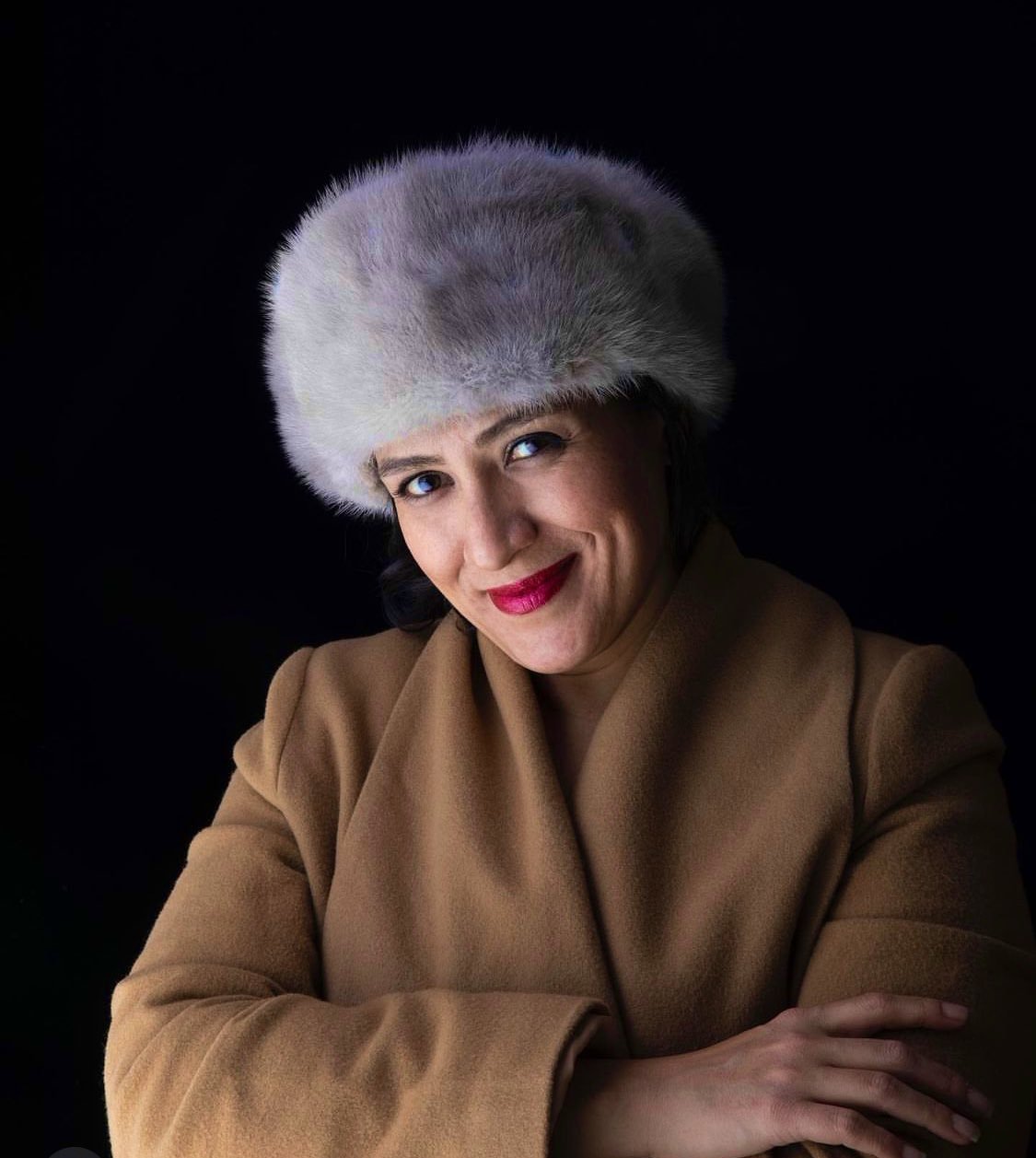The image is a portrait of a Caucasian woman with dark hair and blue eyes, which are partially hidden by a grayish-white fur hat. She is wearing a bright red lipstick and has a genuinely warm smile with a slightly smug expression. The woman is dressed in a camel-colored coat or possibly a trench coat, and her arms are crossed in front of her, with her right hand resting on her left arm. Her head is slightly tilted forward, enhancing her engaging expression. The photograph is softly lit from the lower left, casting a gentle light on her face and upper body. The background is completely black, making her the sole focus of the image.